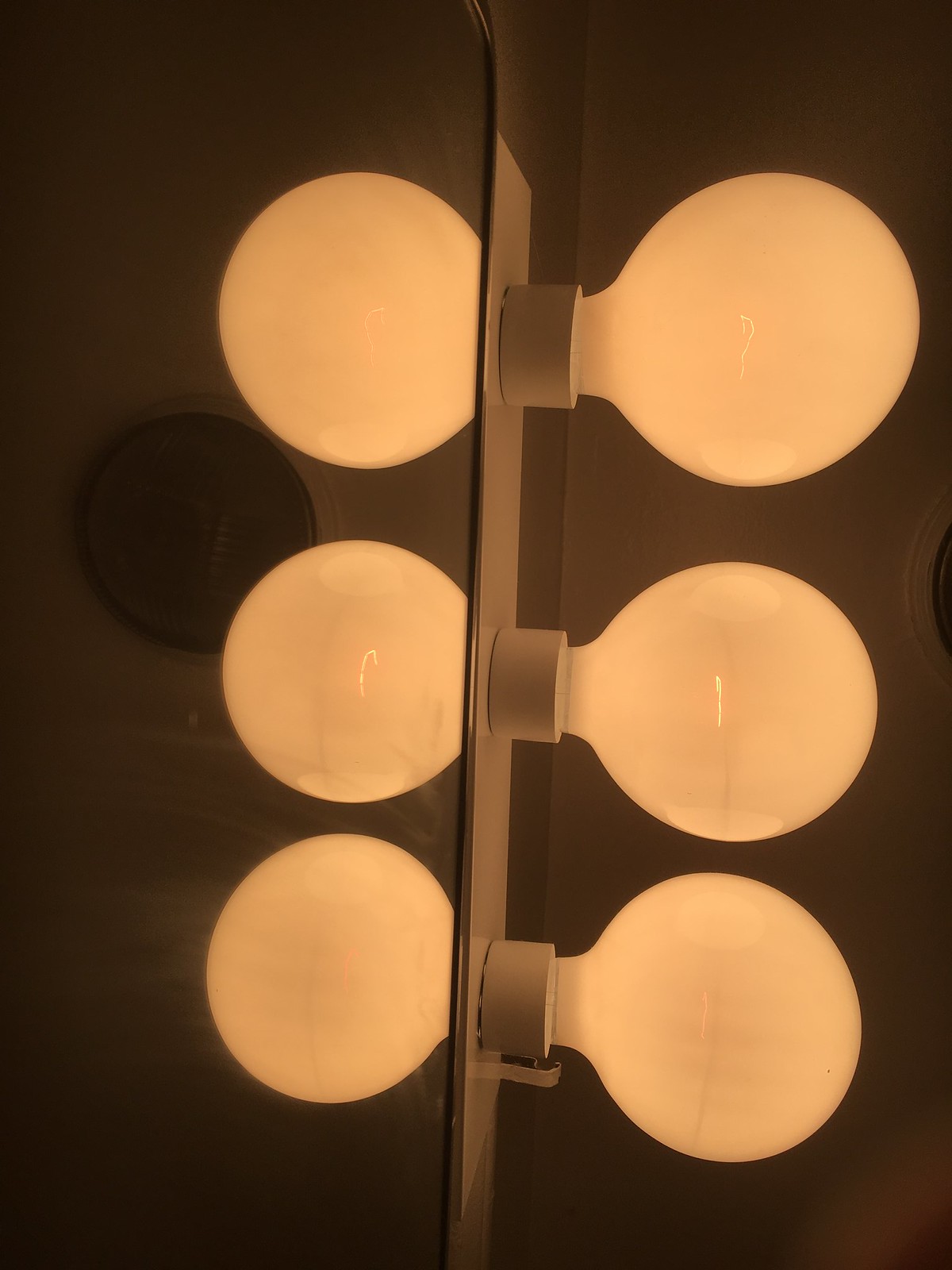The indoor photograph captures a dimly lit bathroom scene. On the right side of the image, three vertically mounted vanity light bulbs emit a warm, yellowish glow, each separated by visible filaments. The background behind these lights is shrouded in darkness, rendering finer details indistinguishable. To the left, a mirror reflects these illuminated bulbs, creating the illusion of six light sources in total. The mirror only reflects the glowing globes and not the sockets, enhancing the repetition of the warm light against the dark background. The photograph, although in focus, retains a low-light ambiance that dominates the overall perception. There is no text or any additional objects visible in the image.